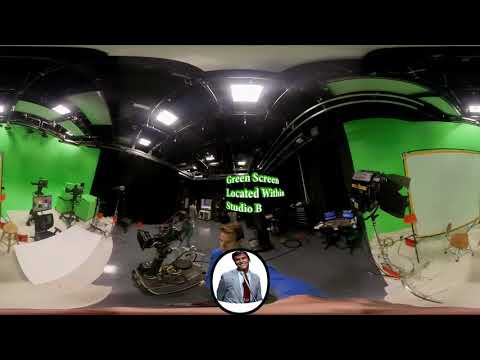The photo appears to depict a television studio, possibly Studio B, characterized by distinctive green handwriting that reads "green screen located within Studio B." The image has a distorted, fisheye lens effect, making the edges appear curved and widened. Prominently visible on both the left and right sides is a green screen backdrop. Black elements adorn the ceiling, including several studio lights arranged in a curved formation.

At the center of the image, beneath the green lettering, a man with short brunette hair in a blue long-sleeve shirt reaches towards the camera. Directly below this, there is a circular frame with a white background, featuring the recognizable figure of Dick Clark. He is grinning, dressed in a gray suit jacket, light blue collared shirt, and a red tie, with a strap across his chest. Notably, the studio setup includes black cameras and metal railings on the ceiling. Overall, the setting and elements suggest a dynamic and busy television production environment.